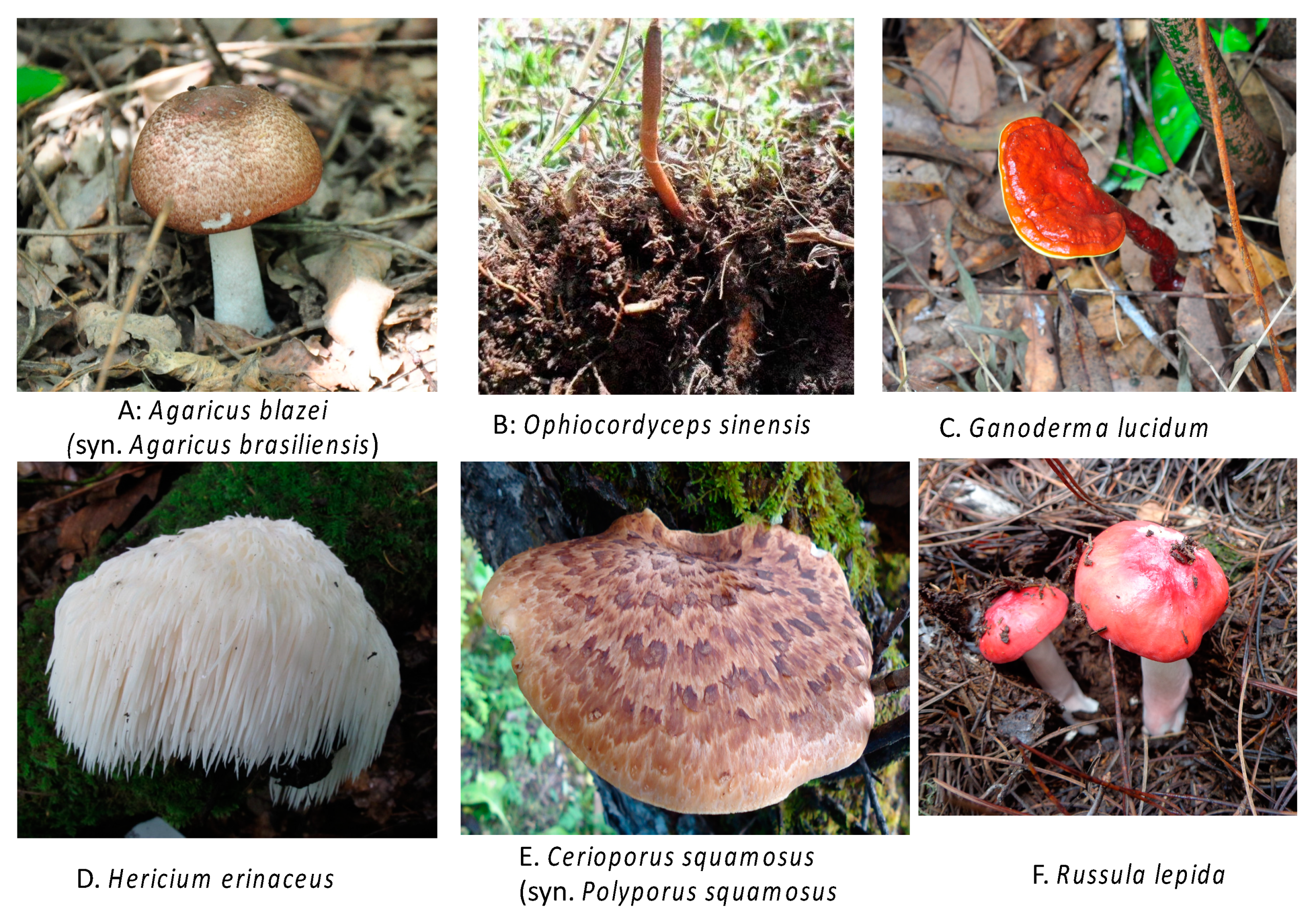The image is a curated collection of six square, colored photographs of mushrooms, organized with three on the top row and three on the bottom row. Each photograph is labeled with both a letter and the scientific name of the mushroom depicted. 

In the upper left corner (A), the image showcases Agaricus blazei (syn. Agaricus brasiliensis), featuring a standard mushroom shape with a brown cap and white stem, situated among dead leaves. The middle top photograph (B) displays Ophiocordyceps sinensis, which resembles a thin, worm-like spike emerging from the ground. The upper right corner (C) highlights Ganoderma lucidum, characterized by its vivid red coloration and slightly slimy appearance, standing out against a backdrop of leaves.

On the bottom row, the lower left (D) exhibits Hericium erinaceus, a mushroom that strikingly resembles a clump of white yarn or a wig of white hair. In the middle bottom (E), Seriporus squamosus (syn. Polyporus squamosus) is presented, showing a large, flat, fan-shaped mushroom with a tan and brown multicolored pattern. Lastly, the lower right corner (F) features Russula lepida, with two mushrooms having classic cartoonish red caps and white stems, reminiscent of the iconic mushrooms seen in Super Mario games.